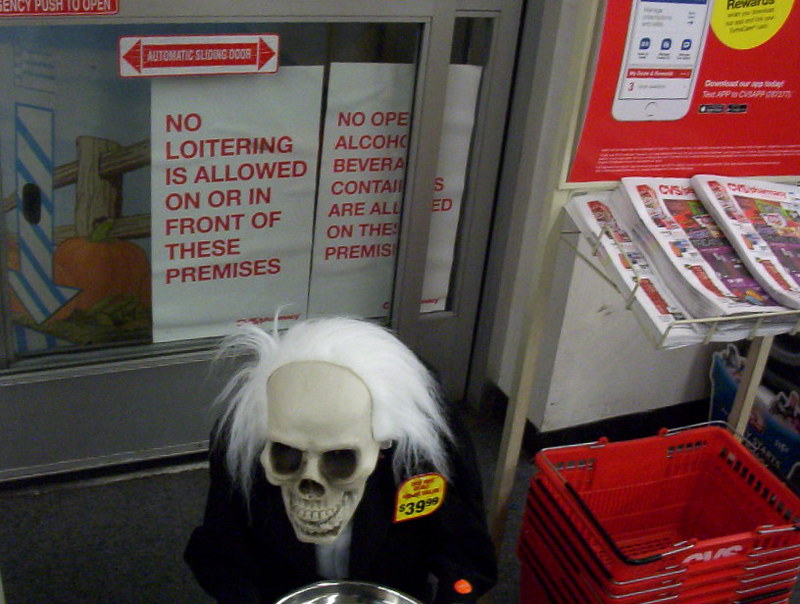The image portrays the storefront entrance of a CVS Pharmacy, adorned with various signs and decorations indicating a Halloween promotion. At the forefront are automatic sliding glass doors featuring multiple notices, including "No loitering is allowed on or in front of these premises," "No open alcoholic beverages or containers allowed," "Emergency push to open," and "Automatic sliding door." These signs are predominantly displayed in red text on a white background. 

In front of the doors, to the right, there is a wire stand holding newspapers above a stack of signature red CVS shopping baskets with dual handles. Adjacent to these baskets stands an animatronic Halloween decoration: a skeleton with long white hair styled in a receding hairline manner, evoking a mad scientist look. The skeleton is clad in a dark coat over a white shirt and holds a silver candy bucket. A yellow price tag attached to the skeleton reads $39.99. There is also a button on the decoration, suggesting it can be activated to make noises.

The doors behind the skeleton are decorated with festive pumpkins and a picket fence, enhancing the Halloween ambiance. The vibrant display and the variety of details clearly signal a seasonal promotional setup at the CVS entrance.